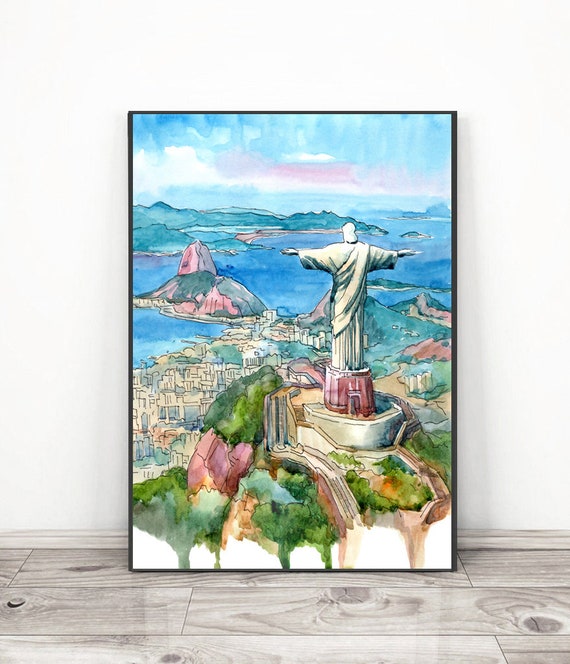The painting depicts a serene island scene dominated by a statue of a robed man with outstretched arms, evoking a Jesus-like pose. The statue, painted in a light gray hue, stands on a white brick platform positioned atop a hill covered in lush green grass. Surrounding the statue's base are reddish-orange rocks, interspersed with vibrant patches of green, yellow, and orange foliage. The statue and hill are framed against a backdrop featuring hints of a tan cityscape with white and tan buildings.

To the right of the statue, additional tan hills are visible, accented by green grass and occasional trees and bushes. Further back, one can see expanses of dark blue ocean, dotted with island-like formations that emerge as dark green hills.

Above, the sky shifts from light blue to white, creating a gentle, almost smudged gradient. Notably, there's a streak of pink that cuts across the center of the sky, adding an unexpected touch of color. The entire scene is set within a painting bordered by a thin black frame.

This framed painting rests against a white wall on a light gray hardwood floor, which appears to be depicted with intricate details such as darker gray lines and grooves, and little circles to imply texture. The floor transitions seamlessly into the wall with a gray strip, contributing to the overall monochromatic ambiance outside the vibrant island imagery. Shadows on either side of the painting suggest it leans slightly against the wall, adding depth to its presentation.